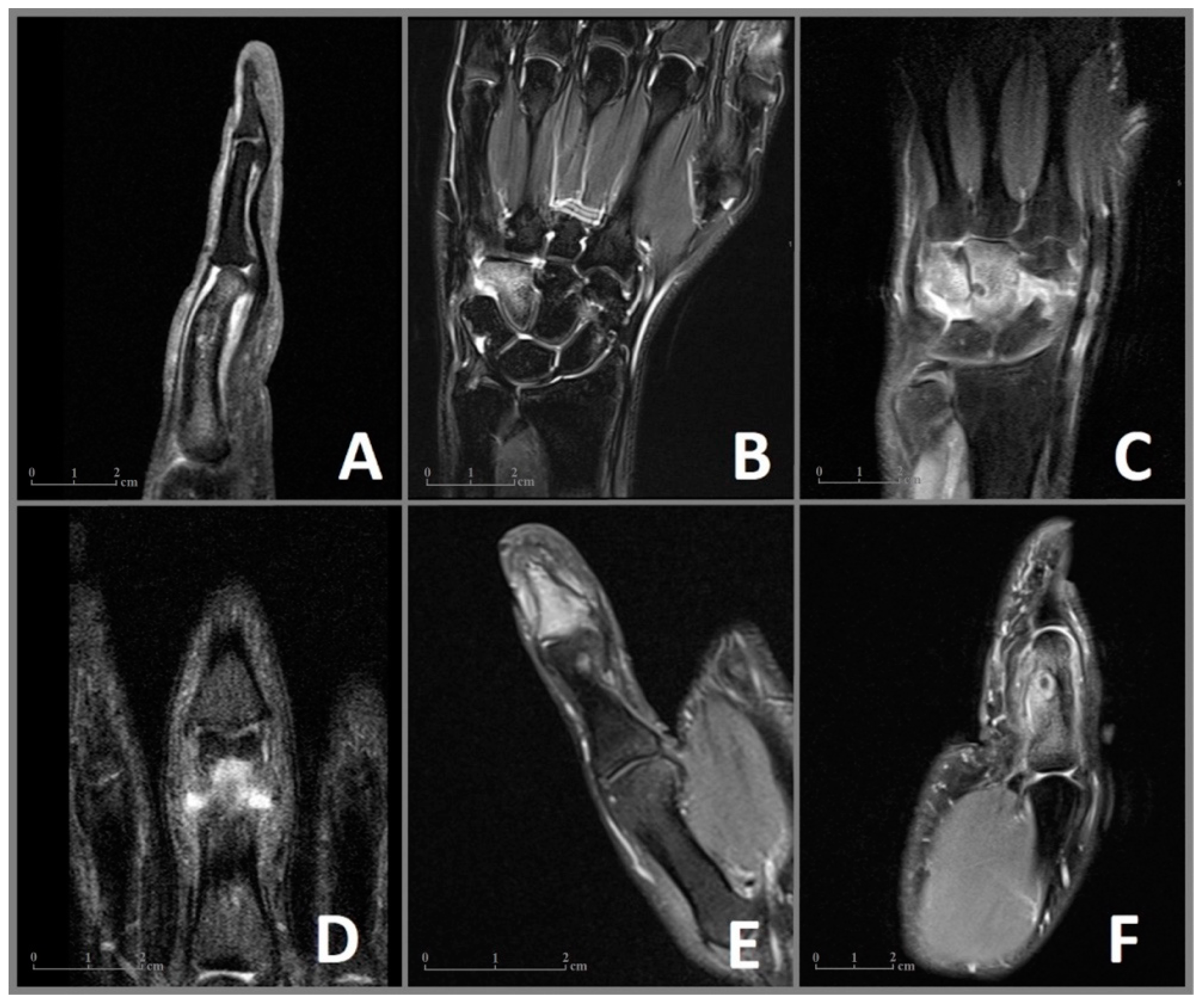The image displays six grayscale images labeled A through F, arranged in two rows of three. Each image appears to depict different parts of a hand, resembling x-rays. Image A, in the upper left corner, shows a side view of a finger with visible phalange bones. Image B, located to the right of A, offers a top-down view of a hand, displaying the bones of an entire hand structure. Image C, in the top right, presents a more ambiguous view but still shows bone-like structures, potentially from the hand or wrist. 

Moving to the bottom row, image D, positioned on the left, focuses on the tips of phalanges, while image E, in the center, clearly shows a thumb with all three bones distinctly visible. Lastly, image F, on the bottom right, depicts a side view that resembles a foot though it lacks clear definition. Each image features a scale on the left side marked zero to two centimeters, offering a sense of size and depth. The overall appearance, in black and white with shades of gray, suggests medical imaging, possibly x-rays or ultrasound, but the peculiar clarity and style might indicate it is not a traditional x-ray technique.